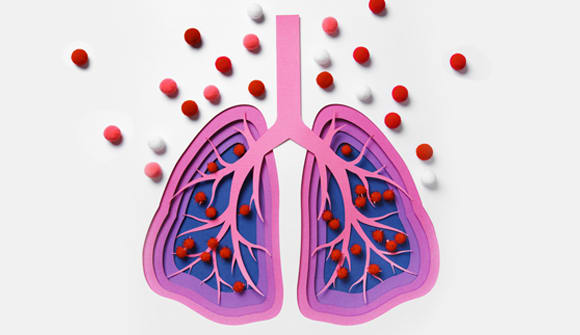This image is a digitally-generated, stylized portrayal of human lungs, depicted with a vivid and intricate design. The lungs are predominantly blue with a network of teal-ish roots branching out from them, enhancing the anatomical representation. Inside the lungs, approximately two dozen red molecules or balls are scattered, likely signifying a harmful substance such as a virus, possibly COVID-19, or other pollutants like blood cells under distress. Outside the lungs, the pattern continues with additional red, white, and pink balls, possibly representing different cell types or further environmental impurities. The vibrant colors and precise arrangement of elements emphasize the invasive impact on respiratory health, making it an evocative visual metaphor for lung infection or disease.